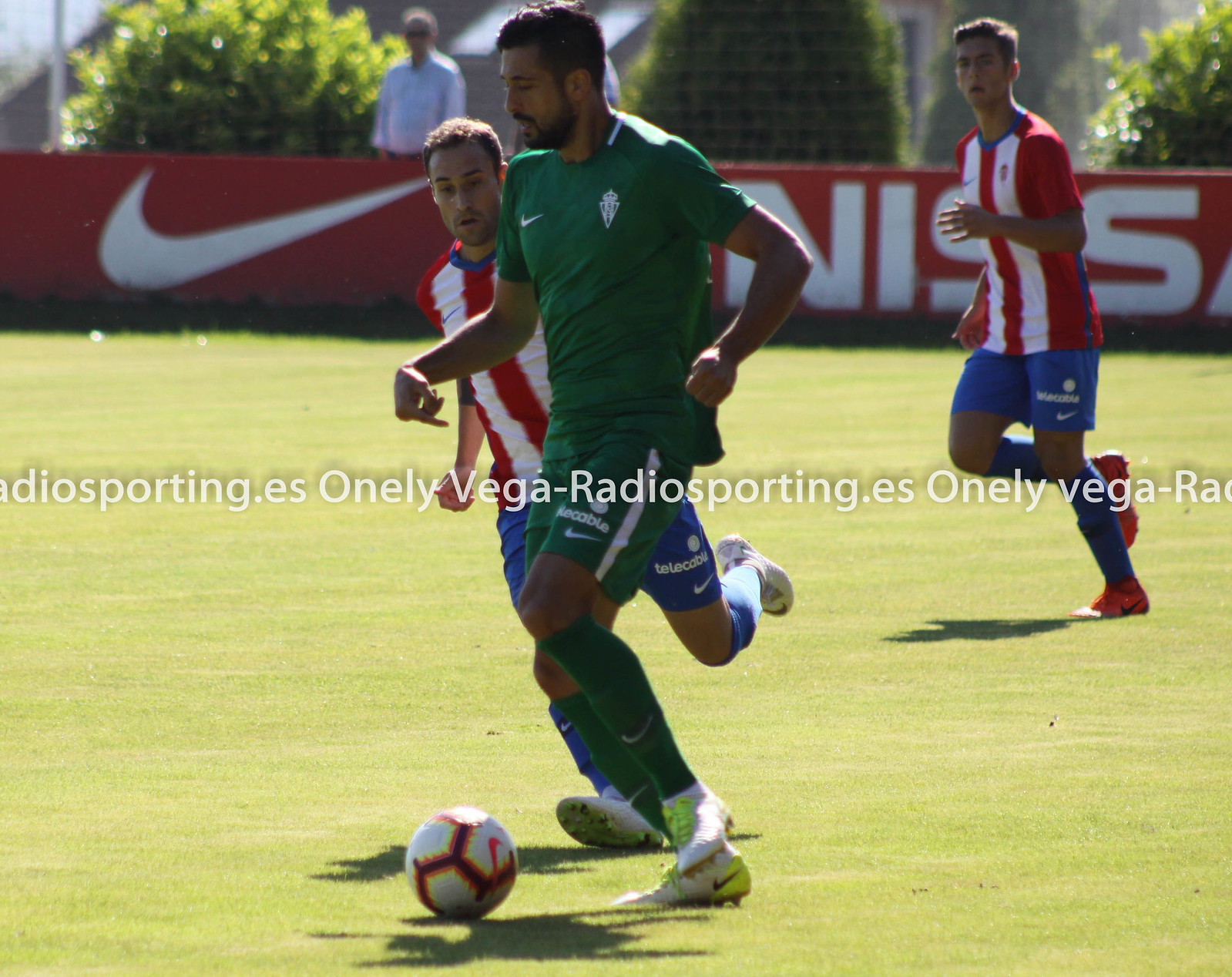In this image from a mid-day outdoor soccer game, a well-manicured grass field spans the scene. Central to the composition are three soccer players in motion: one player in a green jersey, shorts, and socks, likely of Middle Eastern descent, is dribbling the ball. Chasing him are two other players wearing red and white striped jerseys paired with blue shorts and socks. The vibrant colors of their uniforms—green, red, white, and blue—contrast with the green and yellow-tinged grass. In the background, a red wall adorned with a Nike logo and partially obscured text, "Onelli Vega Radio Sporting dot ES," runs horizontally. Behind the wall stands a man in a light blue long-sleeved shirt and sunglasses, observing the game. Flanking the scene are various bushes and buildings, completing the outdoor setting.